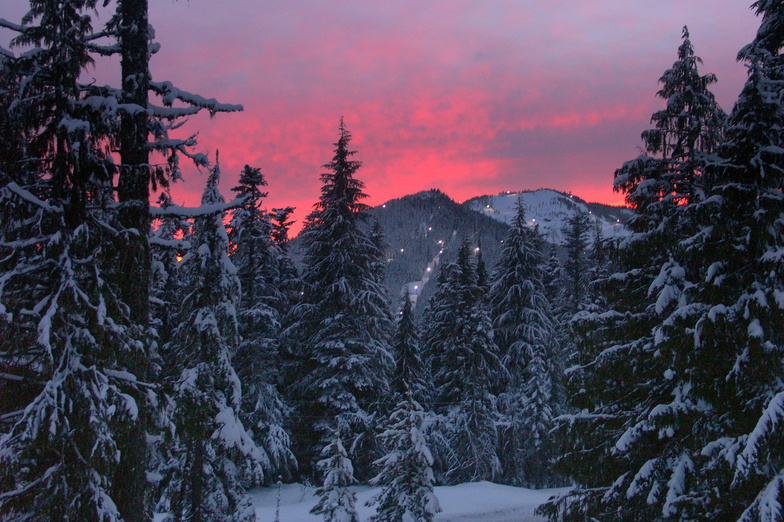The photograph captures a breathtaking winter sunset behind a snow-covered mountain range. The sky is ablaze with vivid shades of red, pink, and purple, juxtaposed against the stark contrast of the gray and black shadows of the towering evergreen trees in the foreground. The trees, both large and small, are blanketed in thick layers of snow, creating a serene and almost monochromatic scene. The ground and tree lines are also covered in snow, adding to the wintry ambiance. In the distant background, the snowy mountain, partially obscured by hazy, fluffy clouds, features faint car lights and possibly a roadway, adding a subtle touch of human presence to the otherwise untouched wilderness. The vivid and fiery sky, coupled with the serene, snow-laden forest, creates a striking and memorable image.